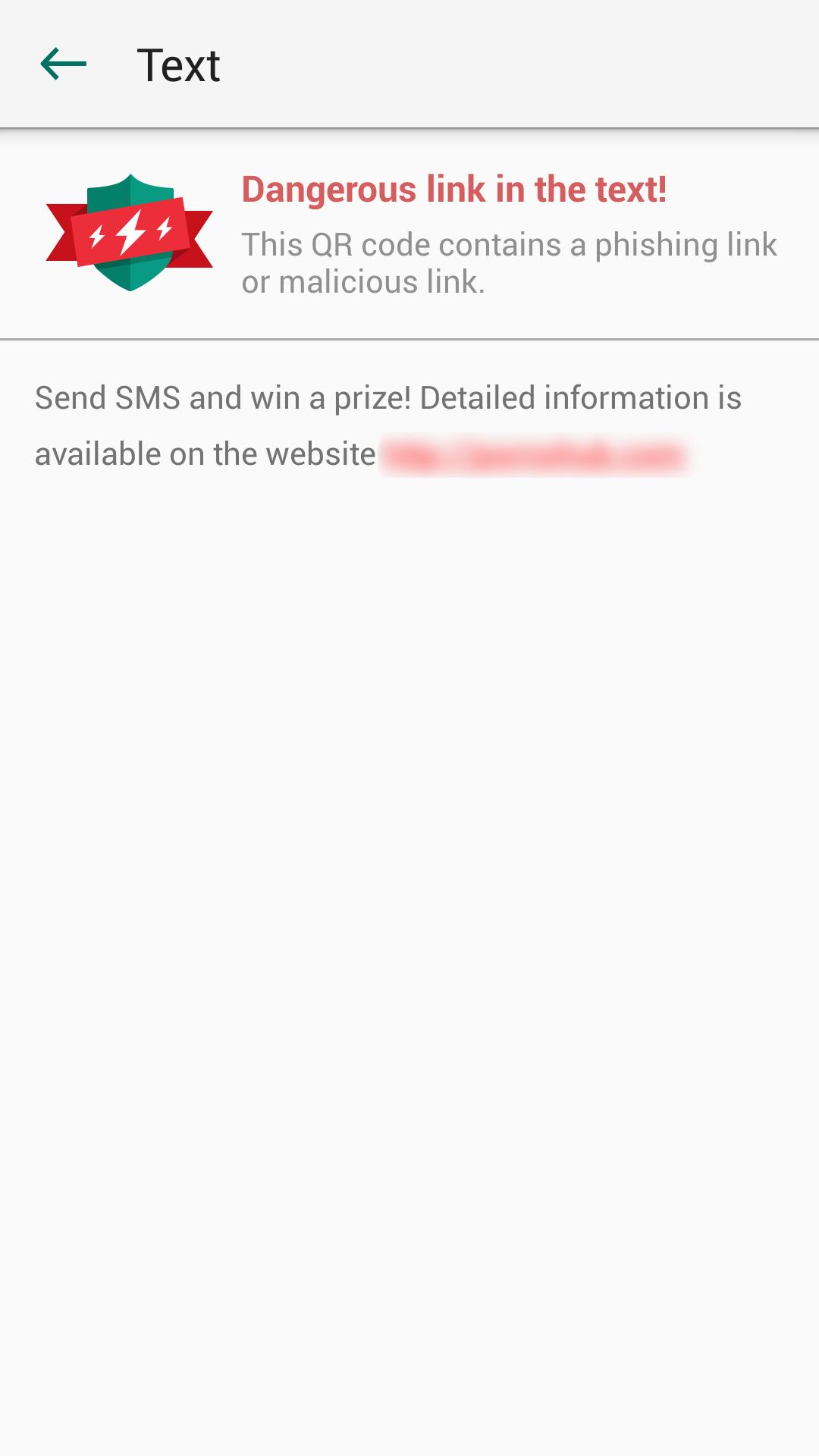The image is a vertically oriented rectangle with a gray background, divided into three sections by black lines. 

At the top of the image, there is a green arrow pointing to the left and the word "TEXT" in black. 

The middle section features a green shield adorned with a red banner and lightning bolts. The red banner contains the text "Dangerous Link" in red letters. Beneath the banner, in black text, it states, "This QR code contains a phishing link or malicious link."

The bottom section displays the message in black text, "Send SMS and win a prize. Detailed information is available on the website," with the website address being blanked out. 

The entire image is set against a gray background without any additional elements.